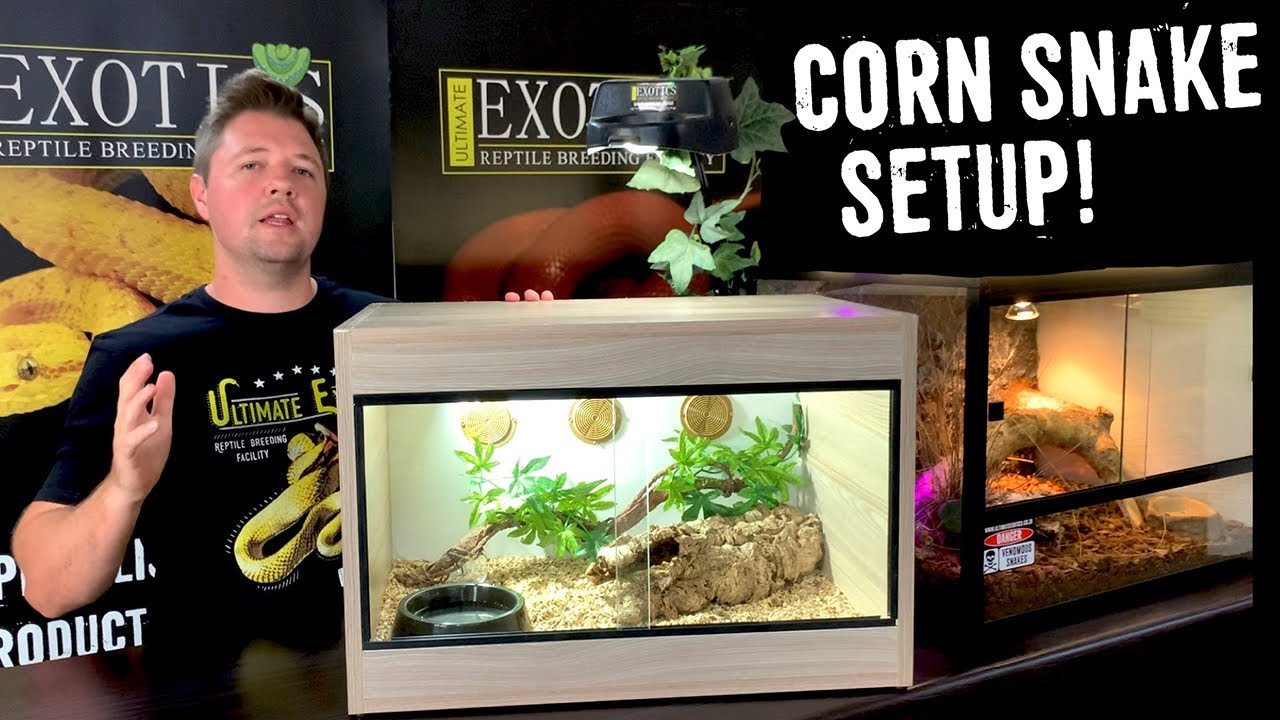The image depicts a mid-30s to 40s white man standing at the center, wearing a black t-shirt emblazoned with a green snake and partially visible text reading "Ultimate Experience for Exotic Snakes." Positioned next to him is a terrarium housing a corn snake, complete with a water bowl, a rock, and some greenery, while another terrarium is seen to the right. The backdrop features a black wall adorned with posters, one of which, located at the upper right corner, prominently displays the words "CORN SNAKE SETUP" in large white capital letters. Another poster on the left side advertises "Exotic Reptile Breeding" with images of snakes, and a logo partially highlighted with the word "RODUCT," suggesting a product-related promotion. This richly detailed scene likely represents an instructional video or advertisement on setting up environments for corn snakes.